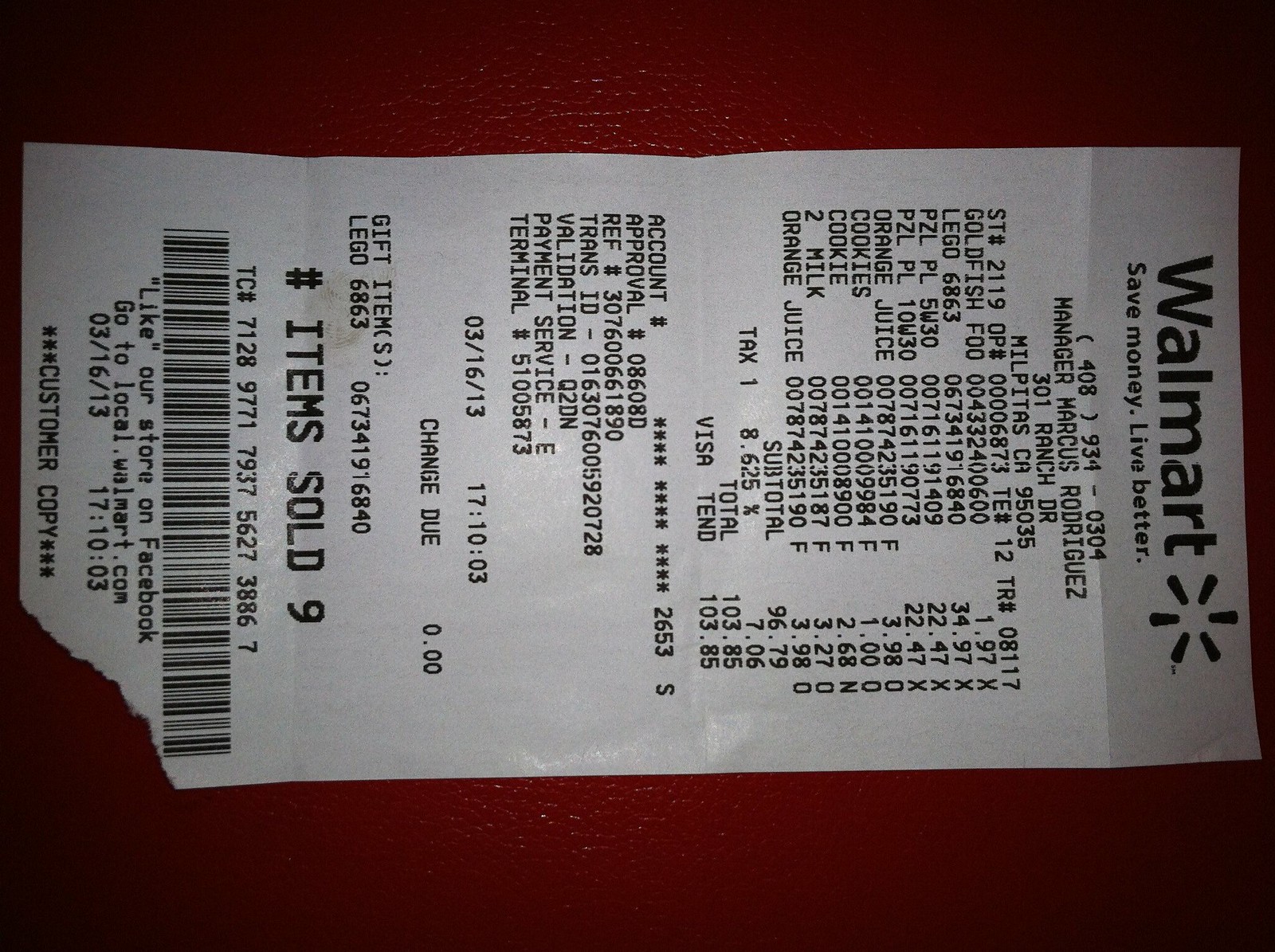The image is a top-down photograph of a Walmart receipt, positioned horizontally with the top directed to the right. The receipt, printed on white thermal paper with black text, lays on a red-colored, shiny surface that is completely flat. There's noticeable vignetting in all four corners, becoming quite dark. The receipt has a small tear at the bottom right-hand corner. Detailed purchases listed include goldfish food for $1.97, a Lego set for $34.97, orange juice for $3.98, cookies for $1.00 and $2.68, and two cartons of milk at $3.27 each. The total amount spent was $103.85 for nine items. The transaction, paid with a Visa card, occurred on March 16, 2013, at 5:10 PM. Additionally, the receipt bears the location of Walmart in Milpitas, California, zip code 95035, and includes a printed gift receipt for the Lego set. The bottom of the receipt notes "Customer Copy" and features a barcode.